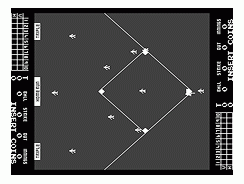The image showcases a close-up view of a retro arcade game screen. On either side of the screen, the words "Insert Coins" are prominently displayed in bold, alongside a series of zeroes (0, 0, 0, 0), likely indicating the remaining credits or scores. The game itself appears complex, featuring a grid-like design with interconnected lines. Within the grid are various small, pixelated figures that resemble tiny people, fish, or airplanes. Additionally, there are several diamond shapes, each positioned in a way that forms a larger diamond structure, with lines connecting these diamonds both internally and to the edges of the screen. A scoreboard is visible on both the left and right sides of the screen, displaying scores or other game-related information. The overall aesthetic and design elements suggest that this is a classic arcade game, though the exact title of the game remains unidentified.